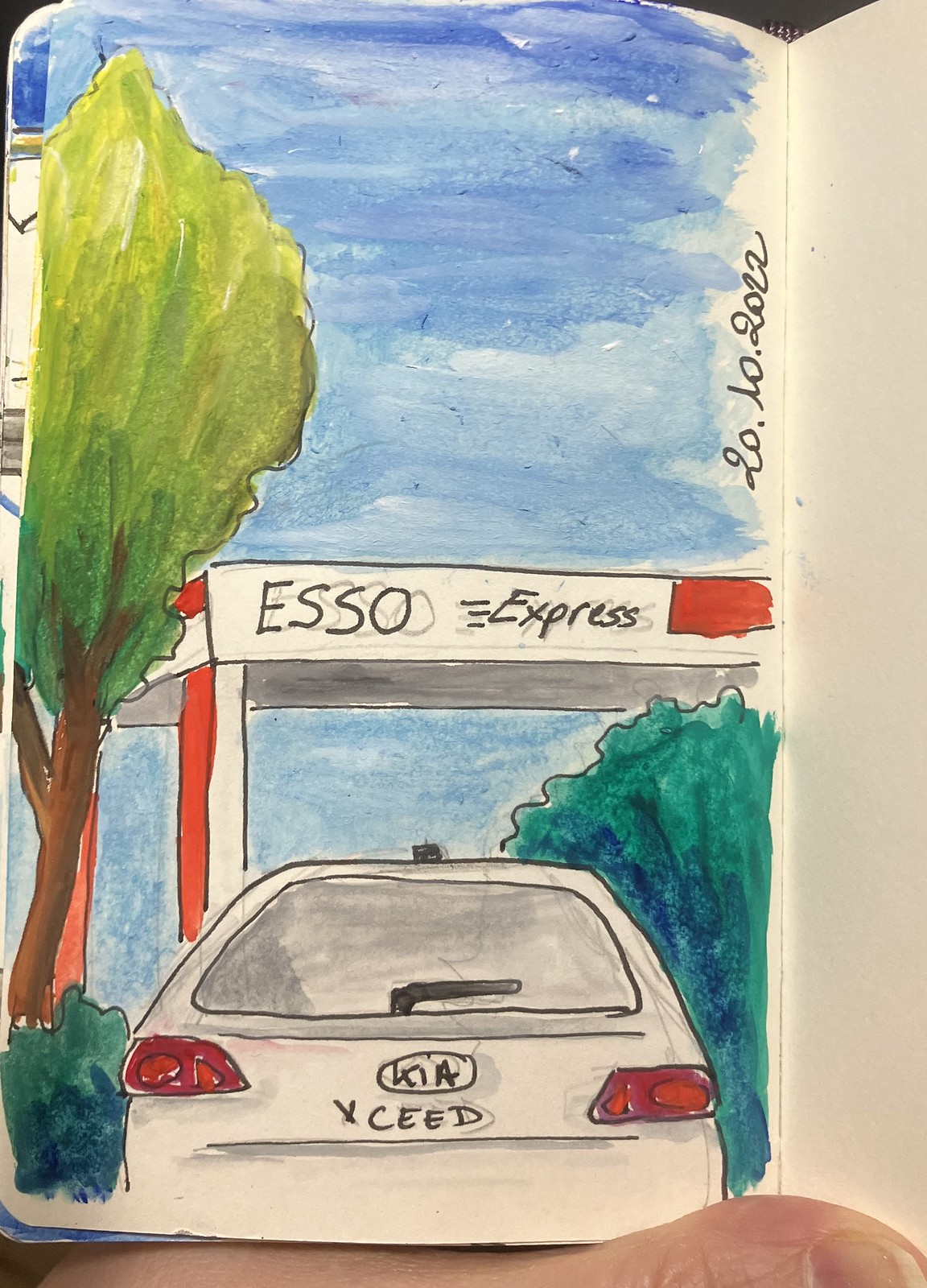This vertical image portrays a page from a booklet, seemingly sketched and adorned with watercolor paints. The composition has an overhead, aerial perspective, with a visible thumb at the bottom holding the page open. The booklet's central crease is evident, alongside parts of the adjacent page to the right.

The page features a watercolor illustration depicting an "SO Express" location, reminiscent of a roadside service or fueling station. A car, resembling a Kia, is shown driving on what appears to be a road, though the exact path isn't clearly defined. Surrounding the car, green trees are painted alongside a blue sky that stretches upwards, creating a serene landscape. The artist has signed their name in black on the right-hand side of the page, completing the scene with a personal touch.